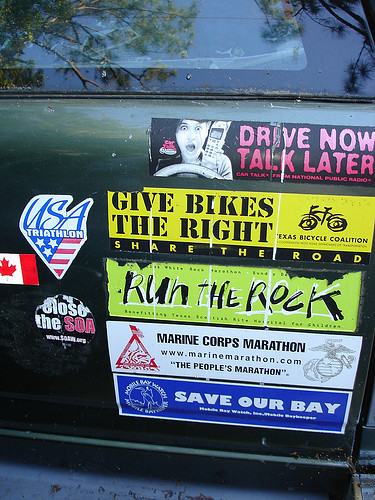The image captures a close-up view of the back of a dark green car, adorned with a myriad of bumper stickers on the lower portion and a window towards the top reflecting a sky and evergreen tree foliage. Dominating the scene is a pink and black sticker at the upper right depicting a shocked woman holding a phone, with the words, "Drive Now, Talk Later," emphasized in pink text on the right side. Below it, a yellow and black sticker advocates bike safety with, "Give Bikes the Right, Share the Road," likely affiliated with the Texas Bicycle Coalition. Beneath this, a green, black, and white sticker reads, "Run the Rock," in stylized text. Further down, a white sticker inscribed in black promotes the "Marine Corps Marathon" and features the tagline, "The People's Marathon," alongside a URL. Below this, a blue and white sticker urging environmental conservation states, "Save Our Bay," accompanied by a logo. To the left, visible stickers include a USA Triathlon logo featuring triangular shapes with U.S. flag markings, a Canadian Maple Leaf flag, and a partially obscured black sticker with white and pink text, saying, "Close the SOA."